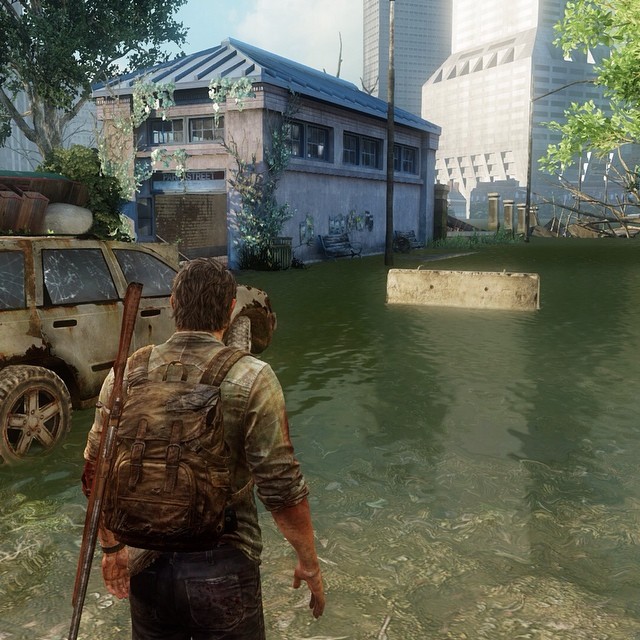This image from a video game presents a highly detailed and realistic 3D rendering of an apocalyptic urban scene in full color. The immediate foreground features a man walking through about a foot of greenish, floodwater, with his back to the viewer. He is dressed in black pants or dark jeans and a greenish or beige long-sleeved shirt with the sleeves rolled up, suggesting an air of practicality and resilience. A brownish-beige backpack is strapped to his back, and a rifle is slung over his left shoulder. His hair is light brown to neck-length, possibly graying, adding to the rugged, survivalist appearance.

To the left and slightly in front of the man, an abandoned vehicle, likely a four-by-four SUV, sits in disrepair, its windows broken and filled with items stacked by former occupants. An adjacent roundhouse-like building or bus station with a blue roof and gray masonry walls adds to the desolate feel, its second-story windows almost obscured by overgrown green foliage. The background reveals more chaos with abandoned skyscrapers and buildings draped in green plants, indicating a long-abandoned, overgrown cityscape. A particularly tall skyscraper stands out toward the back right, dominating the horizon of this flooded municipality. The overall impression is one of post-apocalyptic survival, rendered with meticulous attention to the dilapidation and overgrowth that signify the passage of time in this forsaken urban environment.